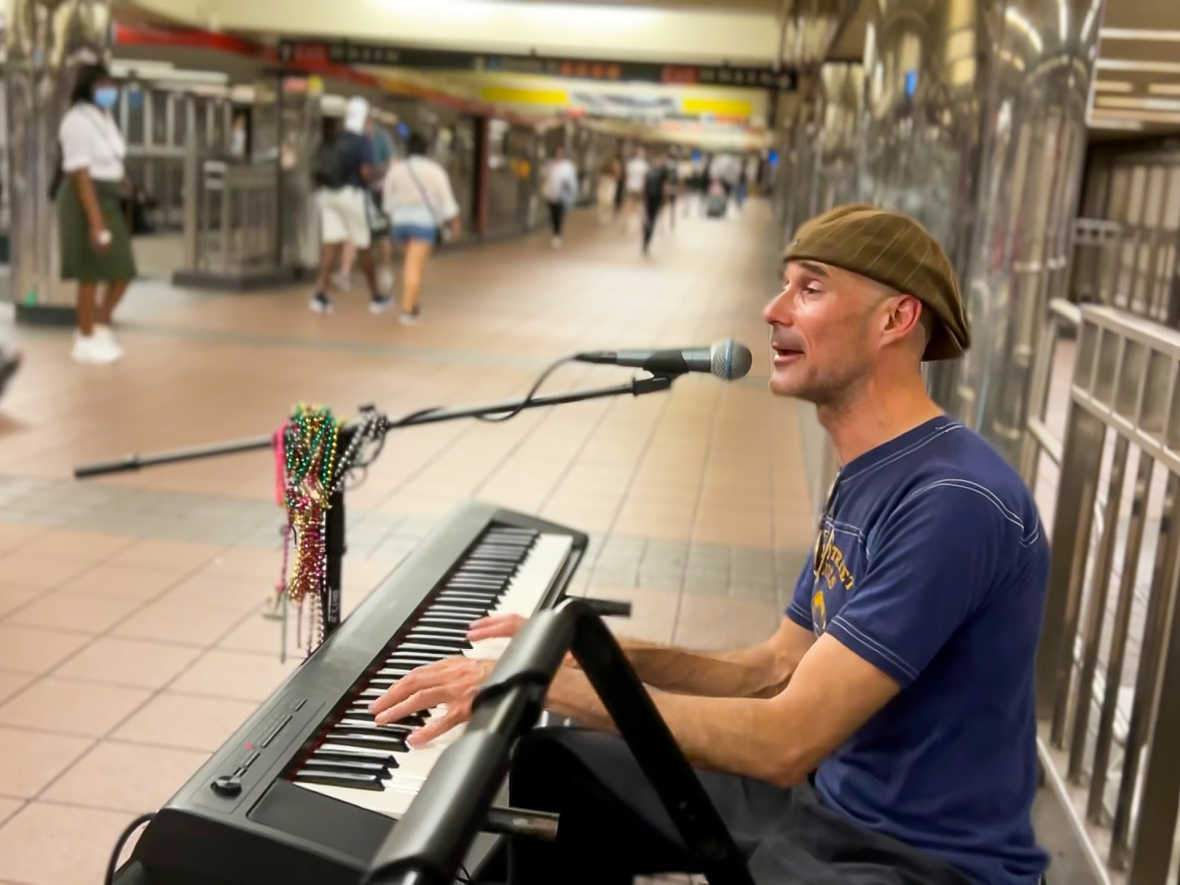In the bustling environment of a New York City subway station, a male street performer captivates passersby with his impassioned singing. Seated on a chair in a corridor lined with square brown tiles, he plays a black portable keyboard. Dressed in a navy blue short-sleeved t-shirt and black pants, he exudes a casual style accentuated by a dark olive green baseball cap worn backward. Peach-skinned with a tanned complexion, the performer appears to be in his 40s or 50s. A microphone, firmly held by his mic stand, captures his every note, while colorful Mardi Gras beads—dark green and dark red—adorn the stand, adding a festive touch to his setup. In the background, the daily hustle and bustle continue, with people walking in both directions and subway signs directing commuters to their destinations. Black signage further indicates the iconic New York City subway lines, grounding the scene in its urban setting.